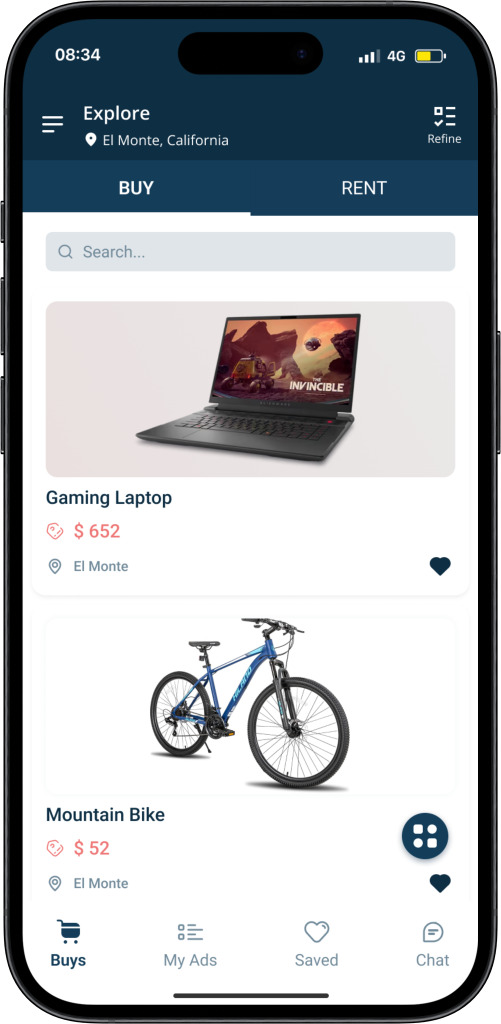The image showcases a black cell phone prominently displayed with all its features visible, including the buttons on the side. The phone's screen shows the time "8:34" on the left side and signal bars indicating "4G" on the right, with the battery icon about half full and highlighted in yellow. Below these indicators, there are three horizontal lines on the left side, indicative of a menu icon. In a line below, text reads "Explore El Monte, California" on the left side and "Refine, then Buy and Rent" on the right side, all in a dark teal blue color. 

The background is predominantly white, with a gray search bar at the top displaying the text "Search" beside a magnifying glass icon. At the top of the screen, there is an image of an open laptop labeled "Gaming Laptop $652 El Monte." Below this, another image shows a blue mountain bike with black tires, labeled "Mountain Bike $52 El Monte." In the area beneath, there are several options including "Buy, My Ads, Save, Chat," suggesting this might be a platform for individuals to sell their used items.

The cell phone specifically displays a screen with the words "I am invincible" set against a space-themed background with an alien spaceship resembling a saucer.